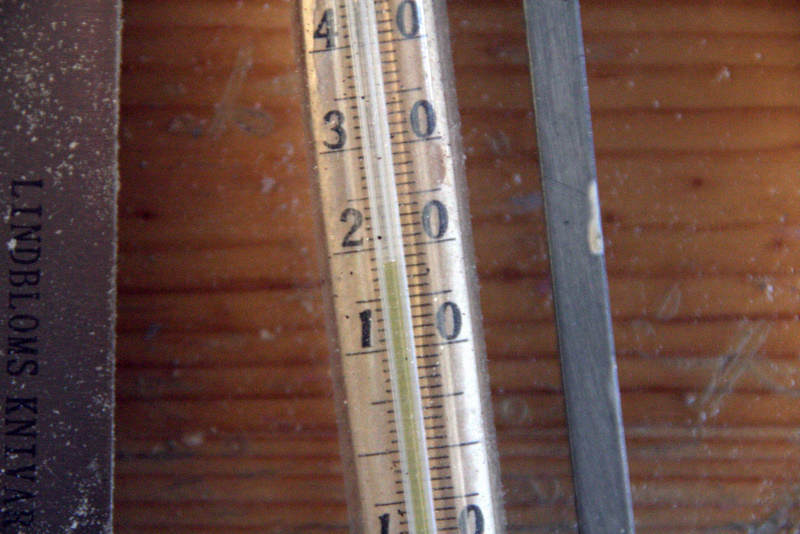This photograph captures a vintage and somewhat worn-out pressure gauge or thermometer, featuring a metallic or light brown metal casing. The focal point of the image is a vertical rod with an attached circular gauge. The gauge displays a reading of approximately 1.8. The gauge's scale on the left side is marked with numbers starting from 1, followed by a space, then incrementing up to 4. On the right side, the scale begins at 0 at the bottom and consists of repeated zeros. 

The background showcases a wood-paneled wall, characterized by its light reddish-brown hue. Adjacent to the device, there is a rectangular black object, resembling a 2x4 piece of wood, with a noticeable patch where beige paint is missing, exposing the material underneath. The overall composition of the image highlights the contrast between the worn metal device and the rustic wooden panel, adding a nostalgic character to the scene.